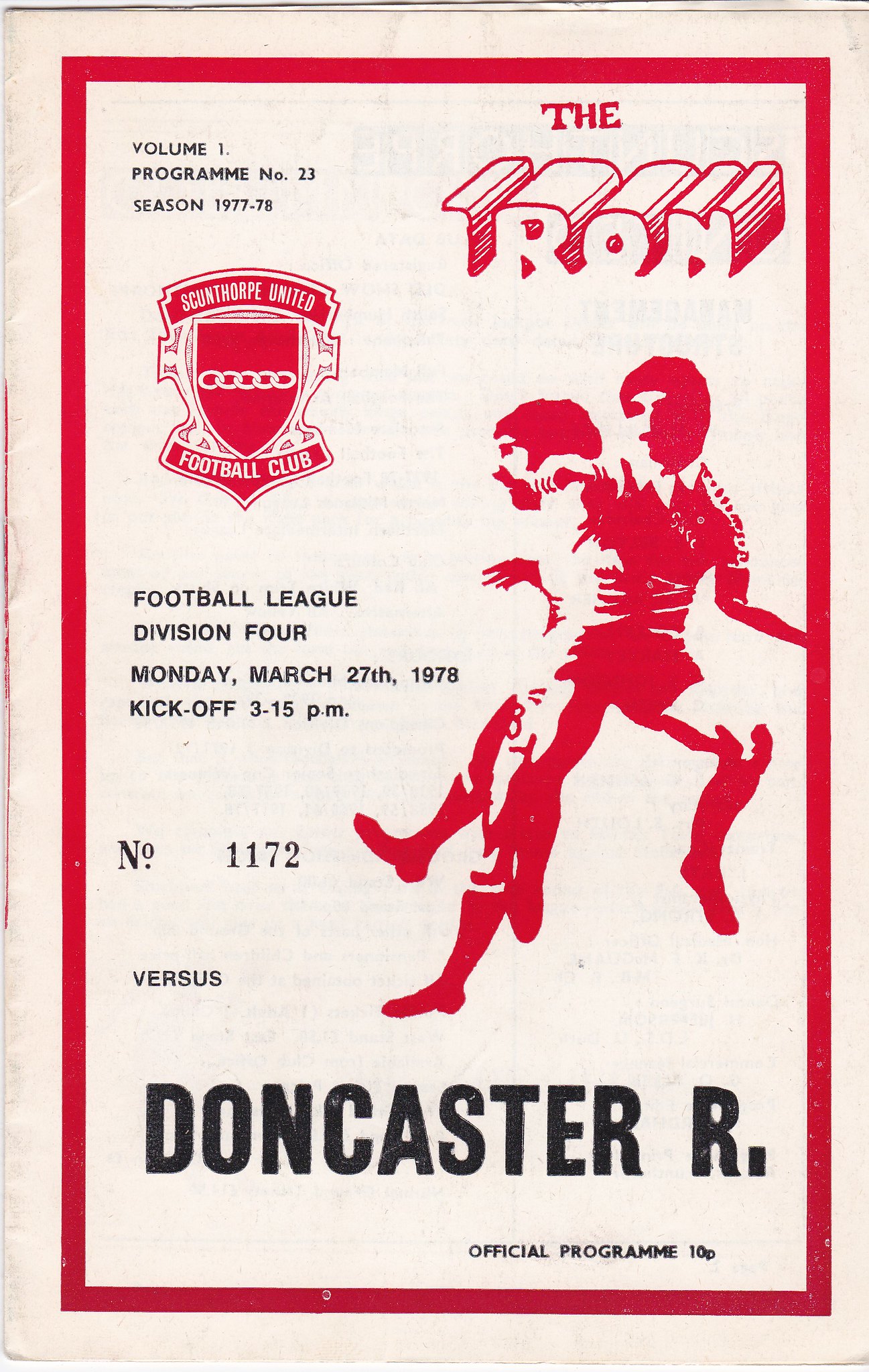The cover of the soccer program, titled "The Iron, Volume One, Program Number 23, Season 1977-78," prominently features text and designs in black and red against an old, slightly creased white background that hasn't yellowed. Displayed in the top section, the program outlines critical information: "Skunthorpe United Football Club, Football League, Division 4, Monday, March 27, 1978, Kickoff 3.15 PM." In the lower region, it is marked "Number 1172" and priced at "Official Program 10 pence." The cover also includes a notable silhouette of two soccer players engaged in on-field action, positioned to the right. Additionally, a shield-like logo with a chain is present, symbolizing the Skunthorpe United Football Club.